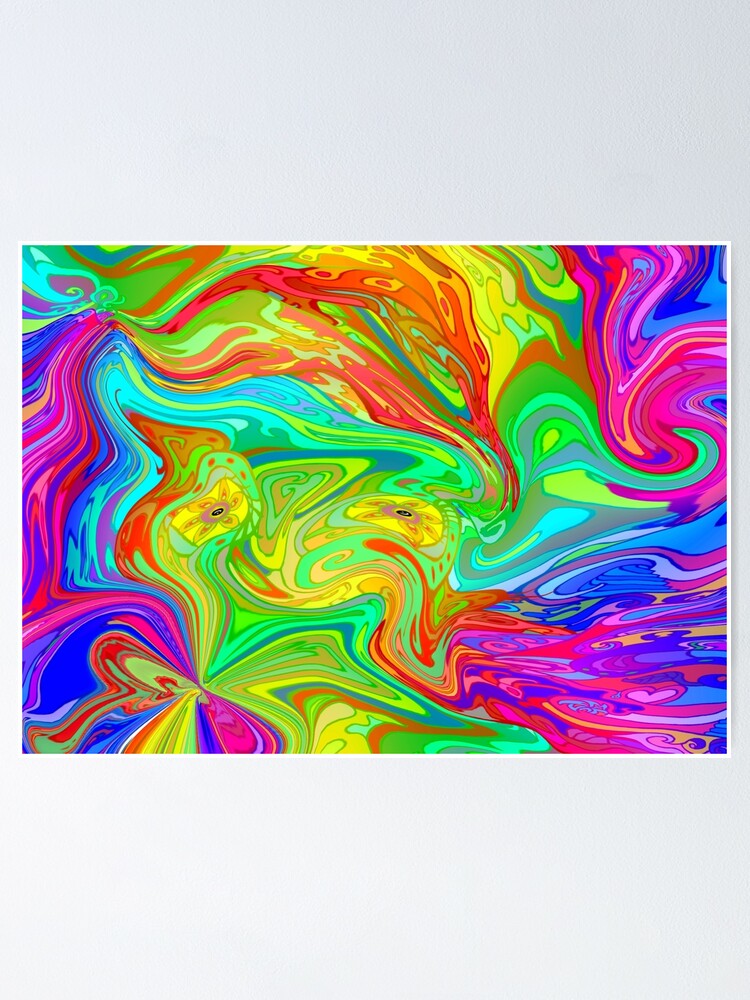The image depicts a vivid and chaotic digital art print of a man's face against a light gray wall. The print is horizontally oriented and features a mesmerizing array of swirly, squiggly lines and abstract shapes, almost as if various paint colors were poured and allowed to flow freely. Dominated by the entire spectrum of colors—greens, yellows, reds, oranges, blues, teals, purples, and pinks—the design resembles a psychedelic tie-dye pattern. Notable details include two distinct yellow circles with a flower-petal-like appearance in the middle, set against a background where colors blend and swirl together, creating an impressionistic face emerging from the chaos. The mixture of colors ranges from a bluish hue with pink and purple on either side to reddish tones at the top and yellowish-green with pink at the bottom. Despite the abstract nature, the eyes are discernible, giving some semblance of structure amidst the colorful, flowing mess. The overall effect is a trippy, colorful, and fluid representation, with no traces of black or white.